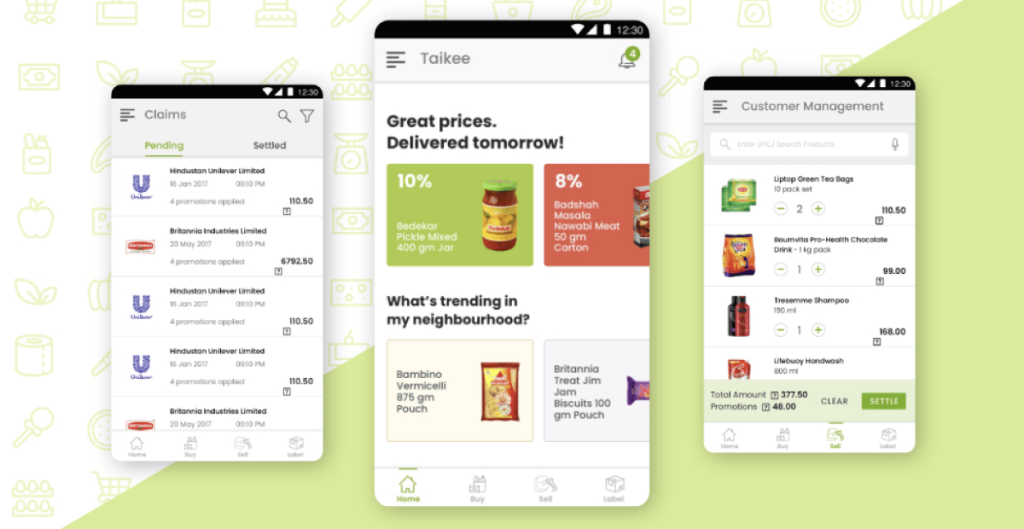Here are three detailed screenshots displayed on a smartphone. The smartphone sits against a visually appealing background, featuring a light green triangle on the right and a minimalist design on the upper-left, which includes light gray icons of apples, leaves, toilet paper, and other grocery items.

### First Screenshot
- **Header**: At the top, in a gray bar, the title "Claims" is displayed. This is accompanied by a search bar and a funnel icon.
- **Tabs**: Below the header, there are three selectable tabs labeled "Pending," "Claims," and "Settled." The "Pending" tab is selected, indicated by a green underline.
- **Content**: 
  - There are five white bars listing different claims.
  - Each bar features a colored icon on the left: three have purple "U" shapes, and two have rectangles containing a red circle.
  - Next to each icon is a bolded description, a date beneath it, and a bolded amount on the right.
  - Amounts listed are $110.50, $792.50, $110.50, and $110.50 for the first four entries. The fifth entry is partially cut off.

### Second Screenshot
- **Header**: Displayed at the top is the word "Talky" along with a bell icon bearing a notification, circled in green with the number four.
- **Content**: 
  - Advertisements for grocery items promoting excellent prices for next-day delivery. The tagline reads "Great Prices Delivered Tomorrow."
  - Featured items include:
    - A pasta sauce in a green-lidded jar, highlighted in a green square with "10%" displayed.
    - Another item in a red square labeled "8%."
  - The section "What's Trending in My Neighborhood" showcases a package of pasta and a candy bar.

### Third Screenshot
- **Header**: The screen is titled "Customer Management."
- **Content**:
  - It displays four grocery items on the left, shown as actual photos.
  - Each item includes a description, the quantity available for selection, and the respective price on the right side.